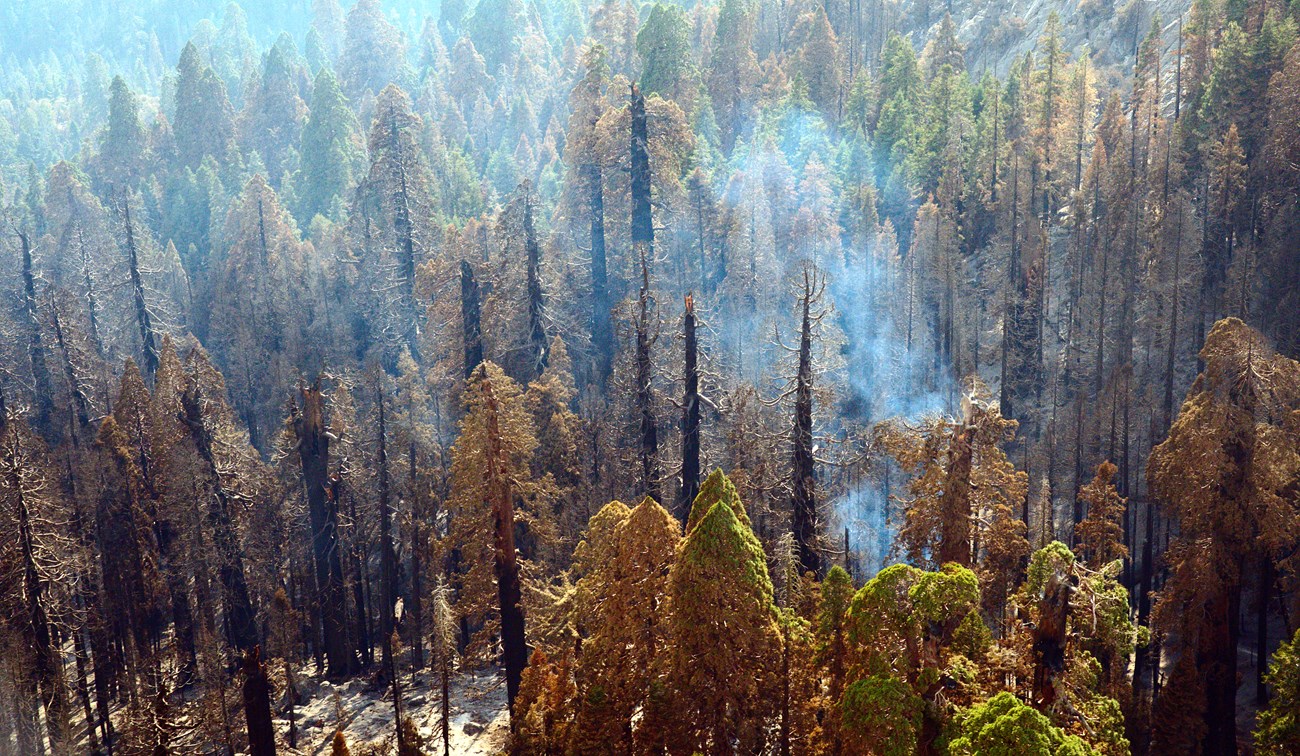This aerial photograph captures a dense and varied forest landscape, with over 100 tall pine trees. The majority of the trees are coniferous, displaying a spectrum of conditions. Toward the bottom left, the trees are sparse and barren, with blackened trunks and no leaves, indicative of damage from a forest fire or other natural disaster. In contrast, the bottom right showcases vibrant green pine trees. In the center of the image, some trees are brown or partially brown, with embers glowing red on the tops, suggesting active burning. A distinct cloud of smoke rises from this area, spreading through the forest. Moving to the background, the forest thickens, and more trees exhibit healthy, green foliage. Bordering the right edge of the forest is a mountain, adding depth to the landscape. No visible life forms such as animals or people are present in the photo.